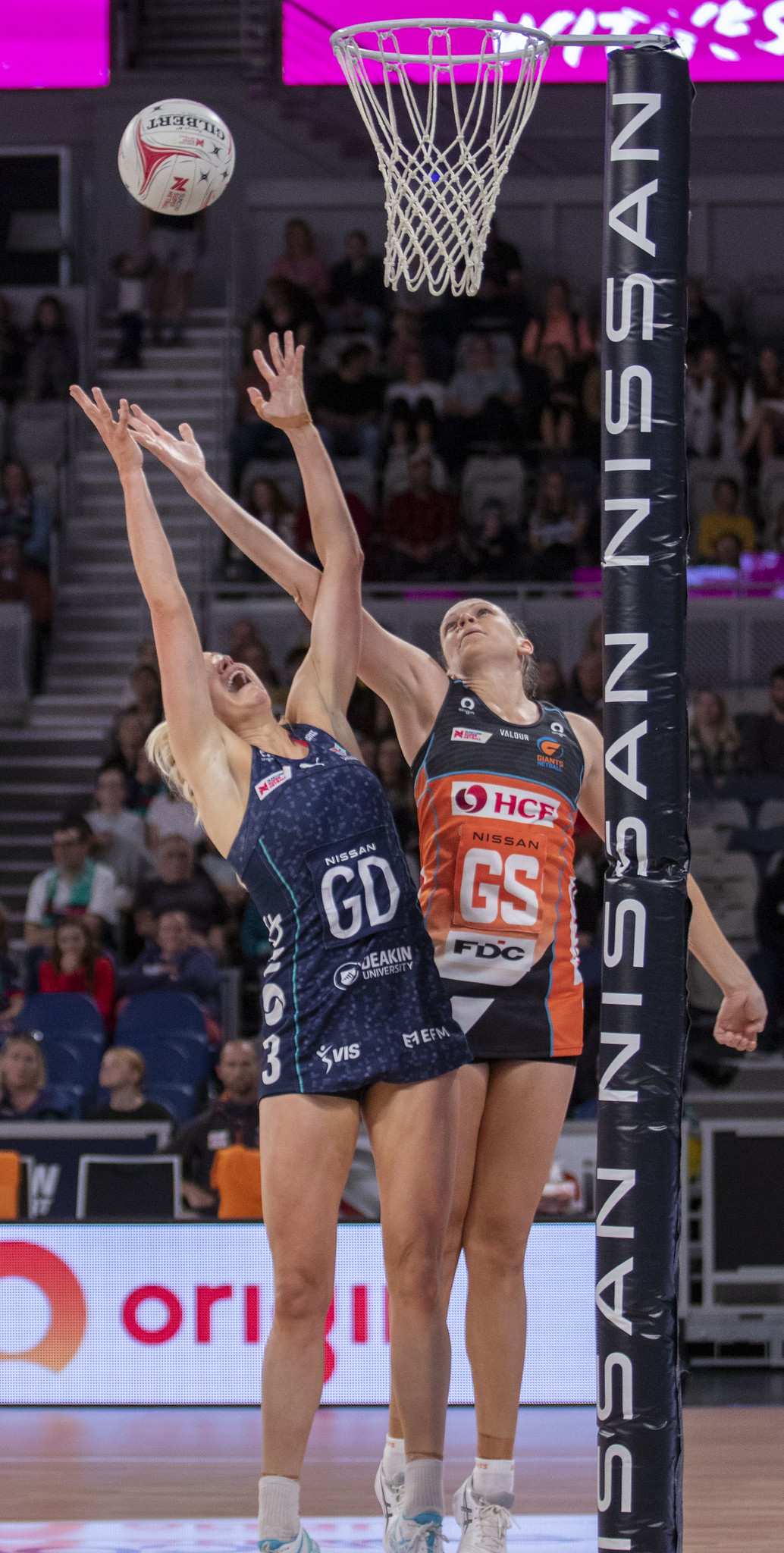The photograph captures a tense moment in a basketball game featuring two female athletes positioned in front of a blue pole with a somewhat rickety hoop attached. The athlete on the left, identifiable by her blonde hair and a blue GD uniform, has both hands extended upwards, presumably defending against her opponent. The athlete on the right, who has dark hair and wears a black and orange GS uniform, is poised with her right hand similarly extended upwards. Both athletes wear long tank tops reaching their hips and white shoes. The ball, which appears smaller than a typical basketball and is colored white, red, and black, is suspended in the air between them. The pole supporting the hoop is branded with the Nissan logo in white on a dark blue cover. The background includes a significant stadium setup with numerous spectators seated on bleachers, along with visible advertisements. Notable among these is a white barricade ad for "Origin" and pink-colored screens displaying advertisements on the upper portion of the photo. The court beneath the players is light brown wooden flooring.